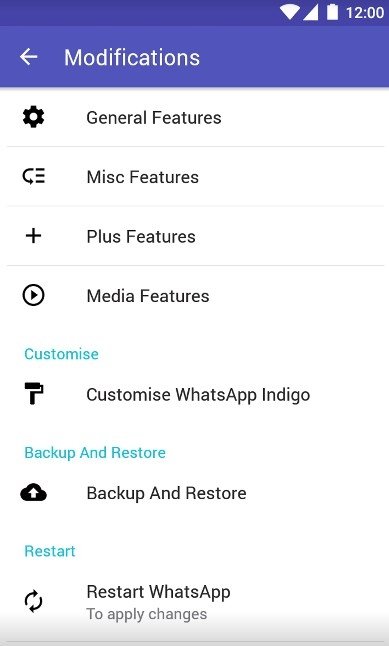A screenshot displays the settings menu of an Android device's WhatsApp application. The screenshot is taken on an Android phone, identifiable by the status bar at the top right, showing it is 12 o'clock, with visible battery level, signal indicator, and Wi-Fi status turned on.

The settings menu is divided into several sections:

1. **Modifications** - A generalized category.
2. **General Features** - Indicated by a gear icon, likely encompassing basic WhatsApp settings.
3. **Miscellaneous Features** - Represented by a three-bar menu icon with an arrow, probably containing varied additional options.
4. **Plus Features** - Depicted with a plus sign icon, suggesting additional features beyond the basics.
5. **Media Features** - No icon detail provided but likely includes options related to media handling within WhatsApp.
6. **Customize WhatsApp** - Details on personalizing the app.
7. **Indigo** - A specific feature or theme, not detailed but distinct enough for its own category.
8. **Backup and Restore** - Expected to cover options for data backup and recovery.
9. **Restart WhatsApp** - An option to reboot the application, typically for troubleshooting or applying changes.

Each menu item is presented in black text on a white background, with corresponding black icons next to the descriptions. The overall appearance is clean and organized, intended to enhance user experience by providing clear, categorized settings options within the WhatsApp application on an Android device.